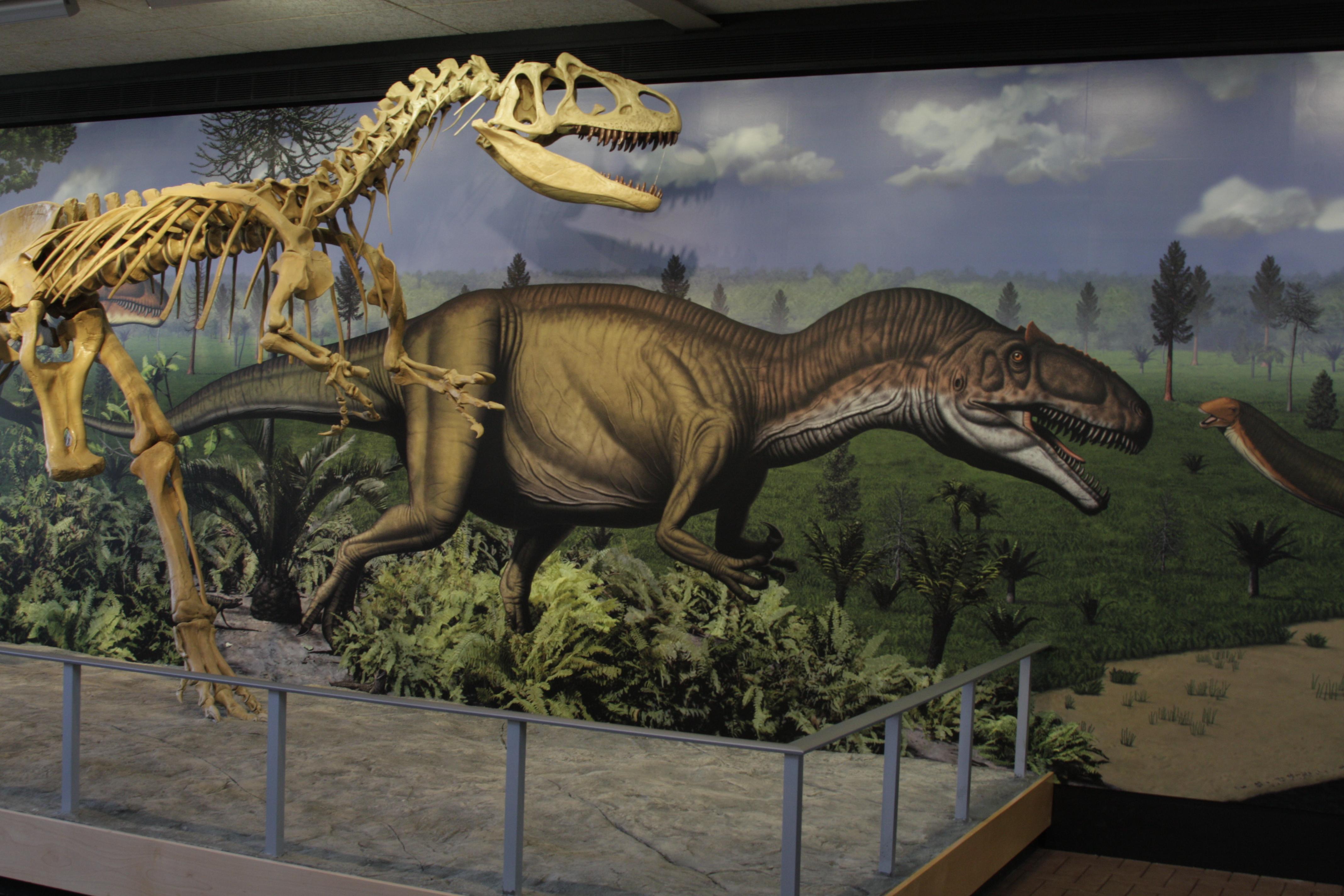This detailed image captures a dynamic exhibit inside a dinosaur or science museum. Central to the photo is a striking display of a T-Rex skeleton, showcased within a secure metal railing to prevent visitors from approaching too closely. This skeleton is meticulously positioned to reflect an action pose, as its open mouth and forward-leaning posture mirror an adjacent mural. The realistic mural in the background depicts a vivid prehistoric scene, featuring a blue sky partly covered by gray clouds, a lush green grass field, and several trees and shrubs. The mural also portrays the T-Rex in the same dynamic stance, providing visitors with a visual comparison to imagine the dinosaur in its natural habitat. Highlighting the exhibit further, lighting accentuates the skeletal structure, offering a close-up view of its intricate bones. Together, the skeleton and the mural create an immersive experience that educates and fascinates viewers about the majesty and scale of these ancient creatures.